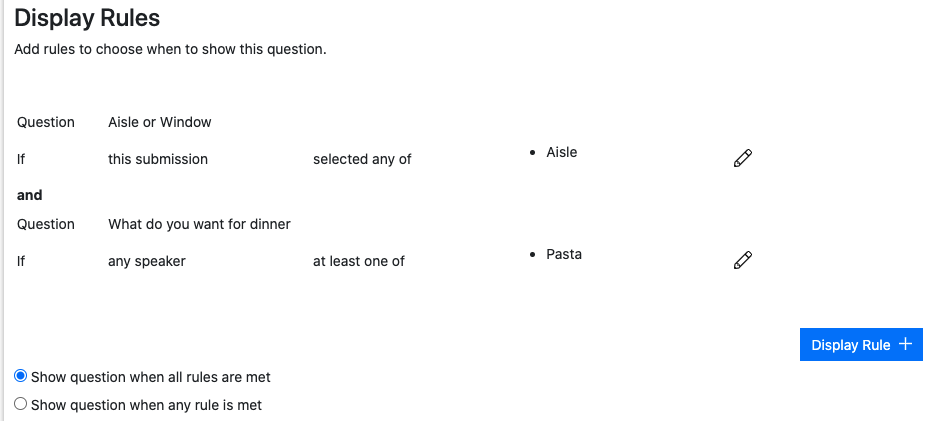This image depicts a web page designed to manage display rules for questions. The interface lacks a URL or specific webpage title. At the upper left corner, the heading "Display Rules" is prominently displayed.

Below this heading, there are sections for specifying conditions to decide when to display certain questions. The first condition is structured as follows: "Question: Aisle or Window?" with a directive stating, "If this submission, select any aisle." Users can interact with this condition, presumably enabling selections via various button options, although the specifics are unclear.

Next, there is another condition labeled: "Question: What do you want for dinner?" This is complemented by the rule: "If any speaker, at least one of pasta." An edit icon, represented by a pencil, appears beside each rule, indicating that users can modify these conditions.

Further down, options allow the user to choose whether the question should be shown when all specified rules are met or when any rule is met. The option "Show question when all rules are met" is highlighted in blue, signifying its selection. Additionally, there is a prominent blue button on the right side labeled "Display Rule +," likely used to add new display rules.

The entire interface is minimalist, featuring a white background with black text and occasional blue accents that denote selectable items and active buttons.